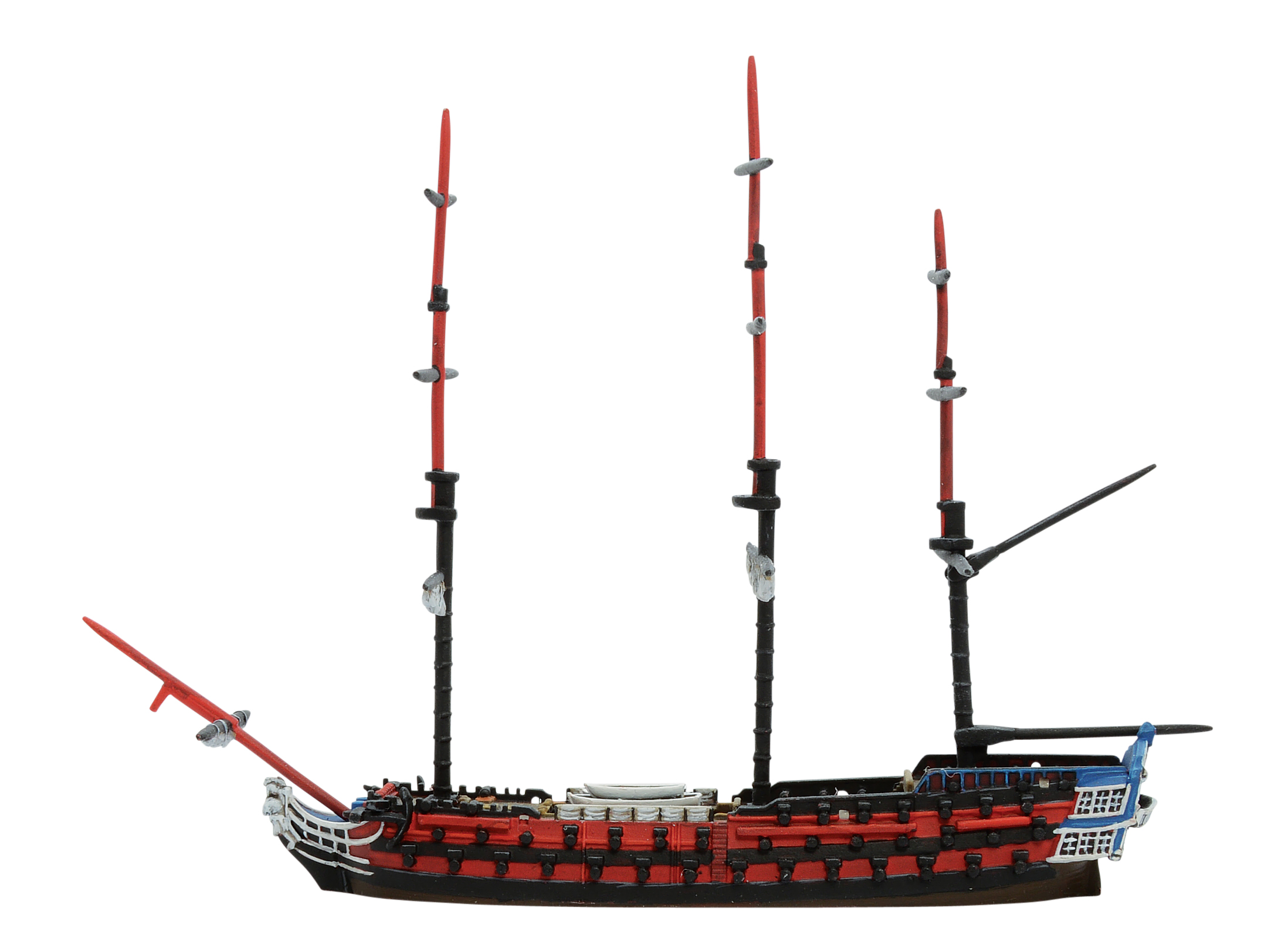The image showcases a meticulously detailed miniature model of a large ship, possibly 3D printed or made of plastic, set against a completely white background. The ship is prominently red and black, featuring three tall masts. Each mast is half black at the bottom and transitions to red towards the top, designed for sails but currently without any. The ship's bow extends with a red board, while the stern has a black board. 

Flanking the sides of the ship are two rows of small red squares on a black background, adding intricate details. At the aft of the ship, there are blue and white windows suggesting cabin spaces or rooms. The deck appears complex with several distinct features: a red missile-like structure at the center, black anchors, and a series of decks and staircases. The description also notes the presence of black and orange stanchions, possibly meant for additional sails or decorative elements. The overall design and color scheme—black, red, white, blue, and orange—add to the realism and intricate craftsmanship of the model.